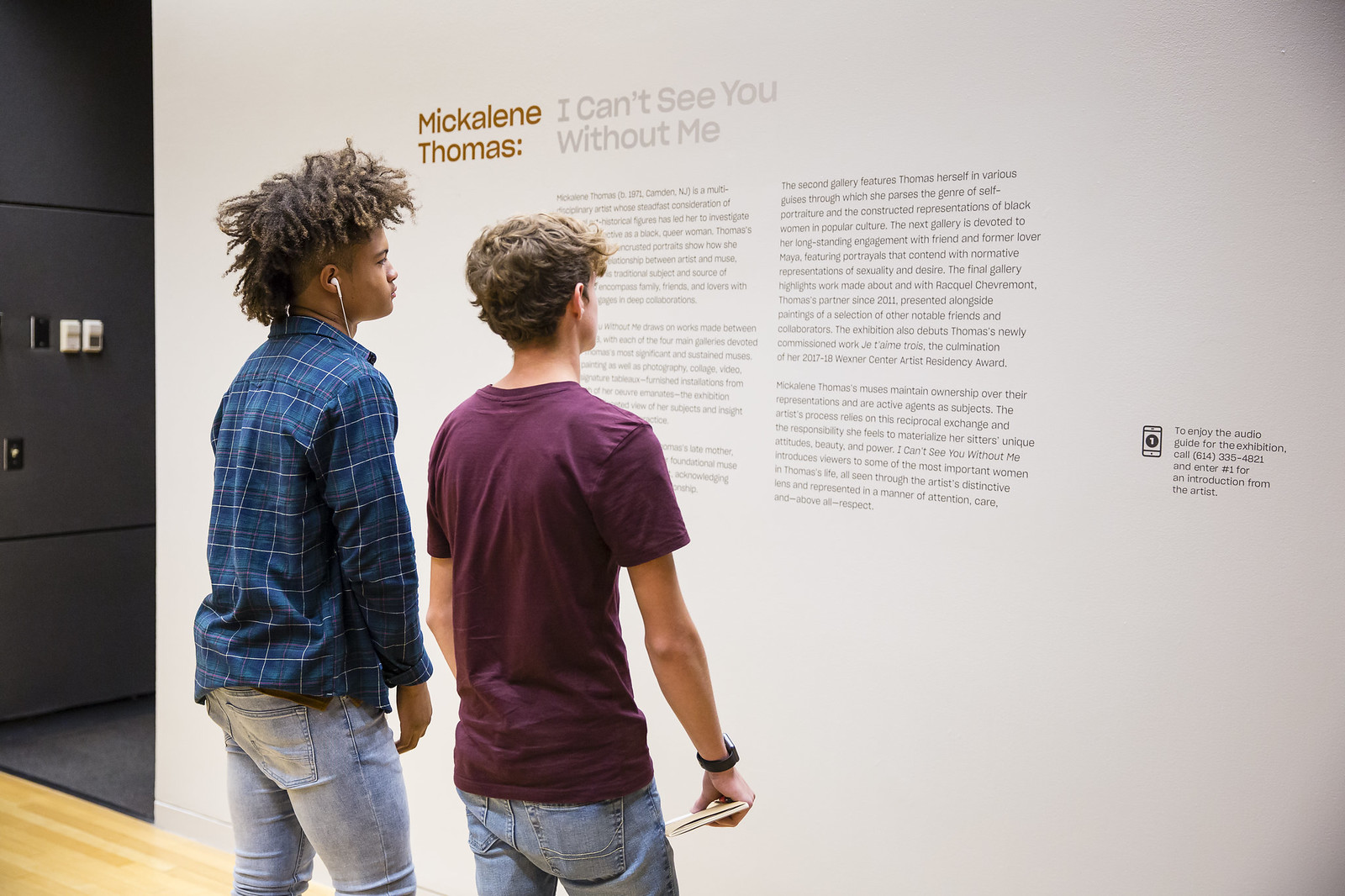The image is a photograph taken in what appears to be a museum or an art exhibit. Centered in the photo are two young male teens, seemingly high school students, standing in front of a textual presentation on the wall. One is an African American teen with short, almost dreadlock-like curly hair, wearing earphones, a blue plaid shirt, and light denim blue jeans. The other is a Caucasian teen with slightly longer hair on top, dressed in a plum-colored t-shirt, a black digital watch, and light blue denim jeans, with a folded pamphlet in his right hand and a wallet visible in his rear pocket. Both youths are intently reading the display titled "Mickalene Thomas, I Can't See You Without Me." The setting includes a wooden floor beneath their feet and a nearby hallway with carpeted flooring. To their left, down the hallway, is a panel and some control boxes on a locked door. On the edge of the wall, a small notification instructs visitors to enjoy the audio guide for the exhibition by calling a provided number. Their backs are turned to us, inviting viewers to share their moment of curiosity and engagement with the art.